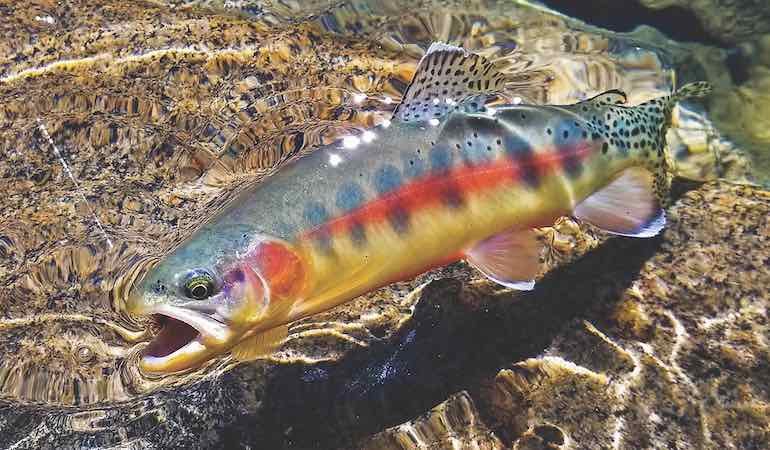This detailed underwater image captures the side profile of a rainbow trout prominently centered in its natural habitat. The clear, rippling water reveals the fish's vivid coloration and detailed markings. The trout displays a grey back adorned with black spots, a distinctive red stripe running from its gill to nearly the tail, and a golden yellow underbelly. Accentuating its vibrant appearance, the trout features purple hues behind its eyes and along oval shapes down its middle. Meanwhile, its top and tail fins are speckled with black. The mouth of the fish is visibly open, possibly with a thin fishing line reflecting from within, hinting at its recent capture. Surrounding the fish, the setting includes tan, yellow, and brown rocks, some forming underwater formations in the image's bottom right, top left, and top right corners. The natural clarity of the water and the detailed depiction of the fish suggest that this close-up photograph was taken by an angler or outdoor enthusiast in a shallow, rocky aquatic environment.